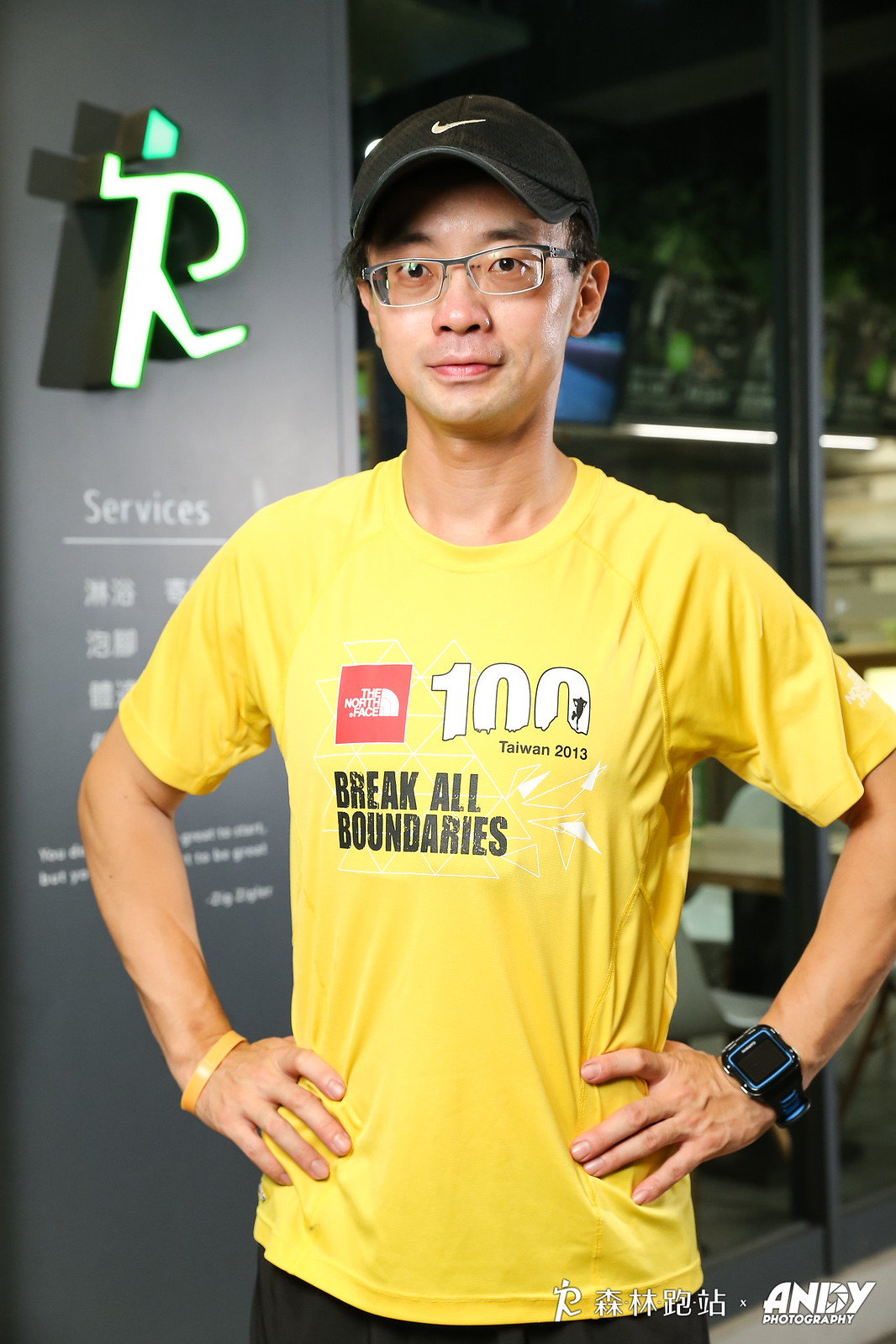This detailed image shows a confident Asian man, presumably Taiwanese, standing indoors. He is wearing a yellow t-shirt that reads "The North Face 100 Taiwan 2013 Break All Boundaries" with an artistic design resembling glass shattering behind the text. His outfit includes black shorts and a black Nike baseball cap. He sports a smart watch on his left wrist and a yellow wristband on his right wrist. The man is posed with his hands on his hips, giving an impression of fitness and readiness, possibly indicating he has just finished working out or training for a marathon. He wears glasses, enhancing his focused demeanor. Behind him, there is a clear background scene featuring a gray wall with a green, illuminated logo resembling a running figure, suggesting a gym or fitness center. The wall also has a prominent letter, possibly an "R", above the word "services" and some Asian text. Additional Asian text and the name "Andy Photography" appear at the bottom right of the image. A glass window in the background hints that the scene is likely within a larger indoor complex, such as a mall.